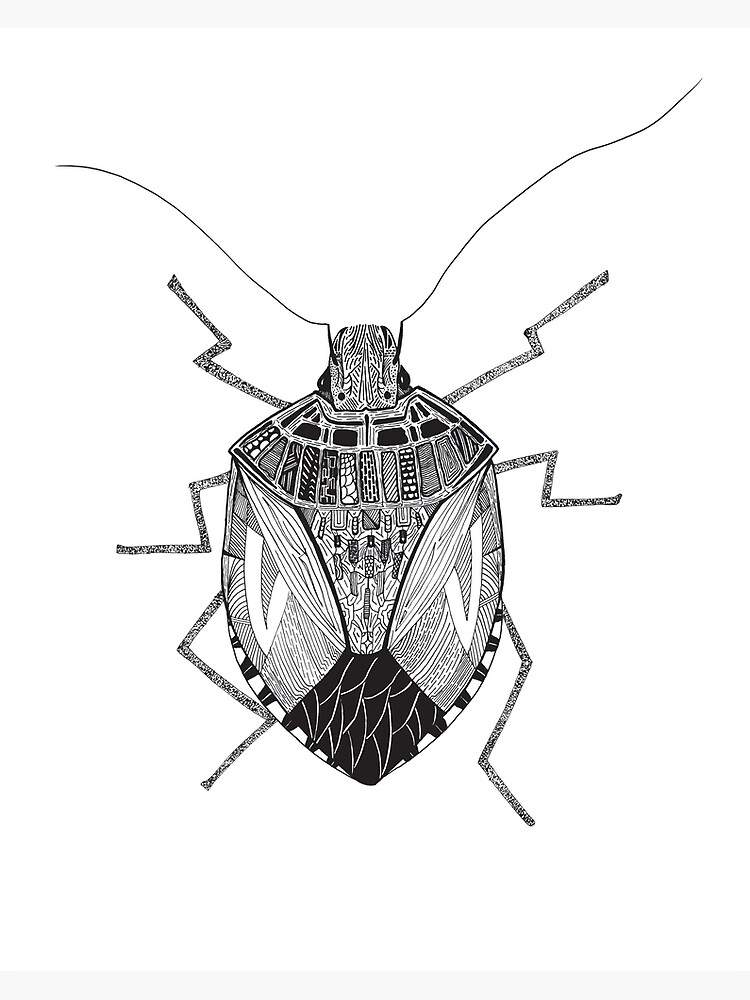This image features a highly detailed, computer-generated illustration of an insect resembling either a beetle or a cockroach. The intriguing patterns and artistic designs on the insect's body make it a captivating subject. Its back displays an array of small rectangles, each adorned with unique patterns, such as brick-like textures and diagonal lines. The insect's wings feature white V-shaped markings, while its lower back area showcases a series of overlapping black shapes reminiscent of wings. The insect has six legs, each depicted as black lightning bolt-like structures splayed out in various directions. It possesses long, black antennae extending from its head and is characterized by small, black eyes. The entire backdrop is a stark white, effectively highlighting the intricately illustrated, monochromatic insect.